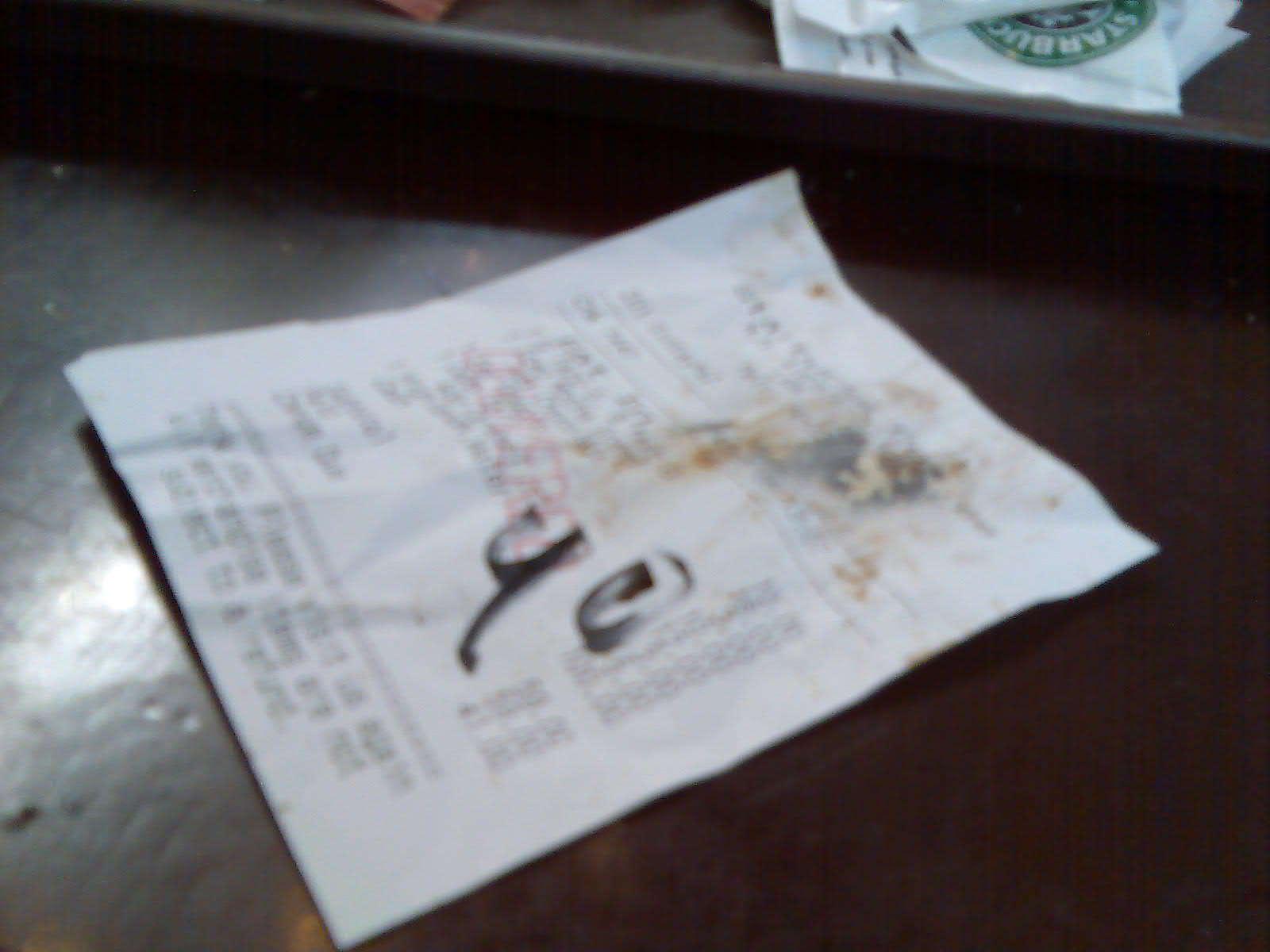The image depicts a blurred photograph of an old, stained receipt marked with a Sharpie, indicating "40" or "90". The receipt is marred by brown dirt and grease stains, suggesting it may have been pulled from an unclean environment. Though the printed text is mostly illegible, remnants appear to indicate several purchased items, with a trace of light red stamping that might denote reserved status. The receipt rests on a finished dark brown wooden table, which has visible dents. Behind the receipt, a gray plastic tray holds a piece of paper with a visible Starbucks logo, characterized by a green circular border and white lettering. The image features no Starbucks products other than this branded paper, possibly a napkin. The receipt dominates the image, with the background elements providing context amidst the blur.